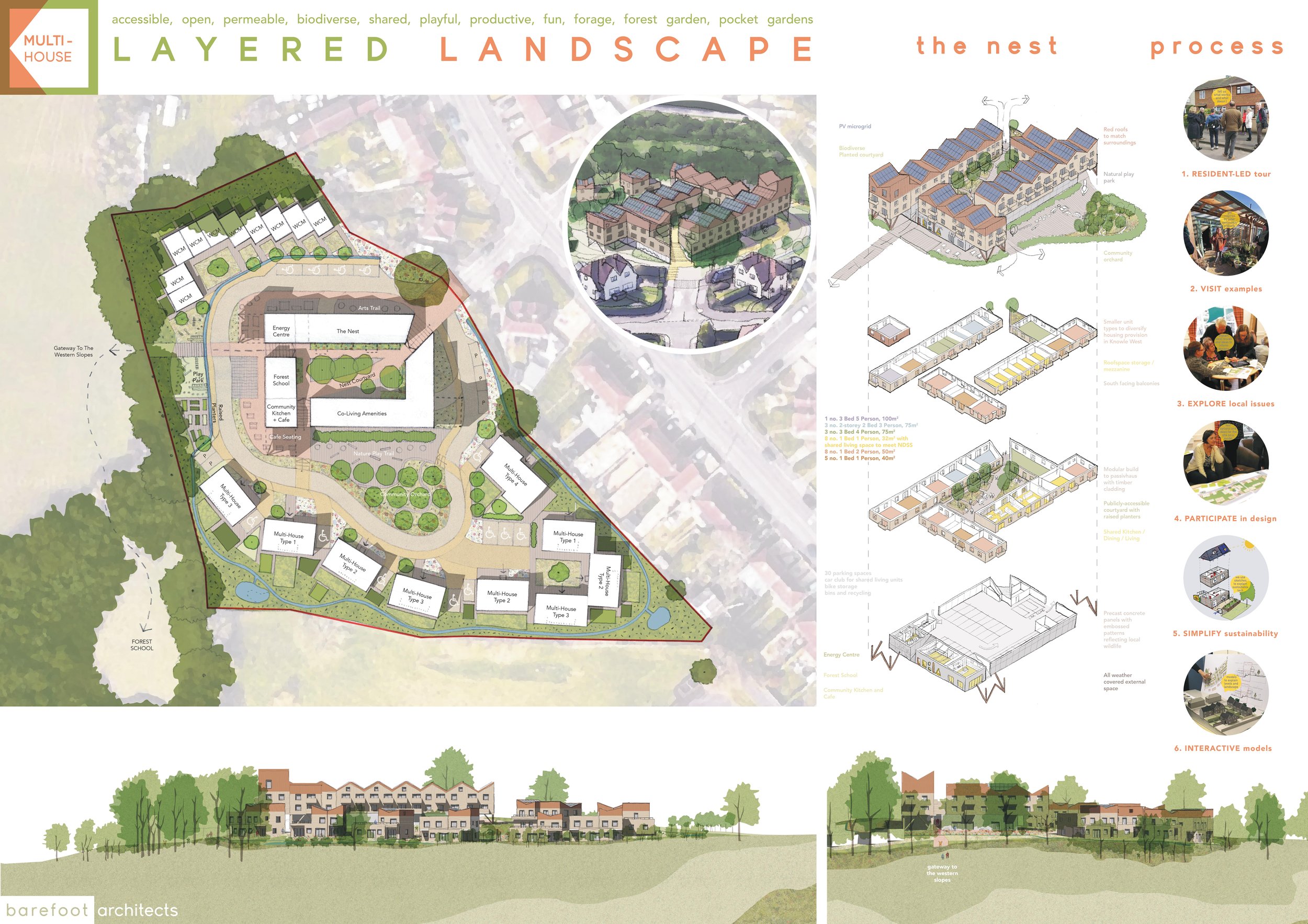The image presents a detailed architectural design for a building project titled "Layered Landscape." At the top, the words "Layered Landscape" are distinctively written in lemon and orange hues. Above this, several descriptive terms, such as "Accessible," "Open," "Permeable," "Biodiverse," "Shared," "Playful," "Productive," "Fun," "Forage," "Forest," and "Garden Pocket Gardens," are highlighted in purple text, emphasizing the project's inclusive and ecological vision.

Adjacent to this, a square logo displays "Multi-House" in bright red letters on a white background with a surrounding box in green, brown, and hints of red. Below the main title, the blueprint reveals the project's structural layout. The right side illustrates detailed sections of the plan, labeled "The Nest Process" in bold red letters. This part of the diagram illustrates various stages of development and community engagement indicated by six distinct processes.

On the lower left corner, "Barefoot Architects" is inscribed, designating the creative minds behind this sustainable and vibrant living space. The detailed imagery includes representations of apartment buildings marked in black, red, white, and tan, surrounded by organized grey streets and housing with grey roofs. Complementing these are green spaces with trees and lawns, enhancing the overall aesthetic and functional quality of the neighborhood.

In summary, this architectural design visually and textually conveys a multi-faceted, community-oriented, and environmentally conscious living space, cohesively blending modern housing elements with natural landscapes for a productive and playful environment.